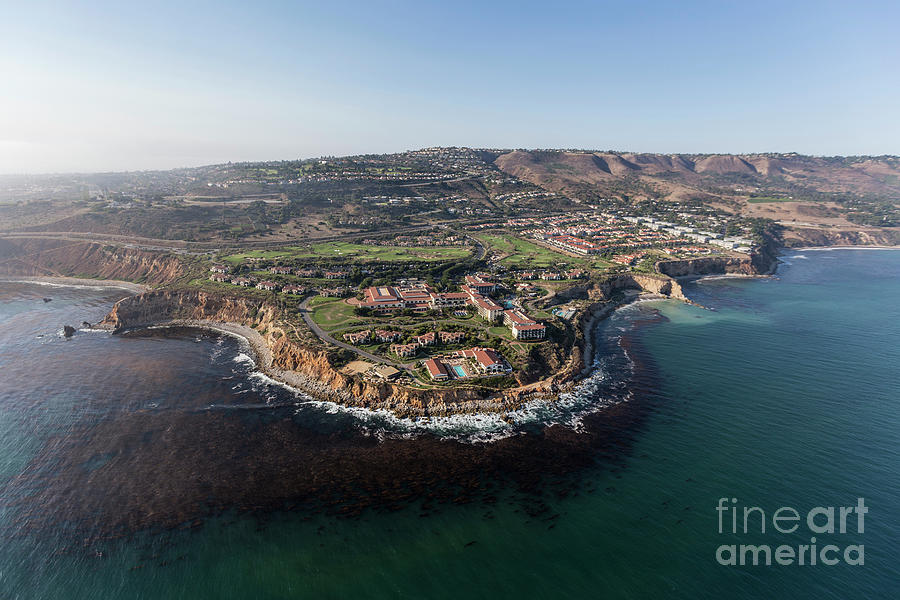This is an aerial photograph from Fine Art America of Rancho Palos Verdes, California, showcasing an expansive coastal resort on the Pacific Ocean. The image presents a detailed view of the entire stretch of the resort, featuring multiple large buildings and several swimming pools, prominently a large rectangular pool in the center. To the right, there's a more populated area with numerous Spanish-style homes, suggesting a wealthy neighborhood. The landscape transitions from the bustling resort and town area to a lush, green, grassy expanse on the left, dotted with cliffs and elevated terrain. The varied topography includes a mountainous range in the background, contributing to the picturesque scenery. A road can be seen leading from the center of the resort down to the vibrant blue, turquoise, and sea-foam green waters of the coastline. The sky is clear, blue, and indicative of a pleasant daytime, enhancing the resort's serene and exclusive ambiance. Text on the image reads "Fine Art America."